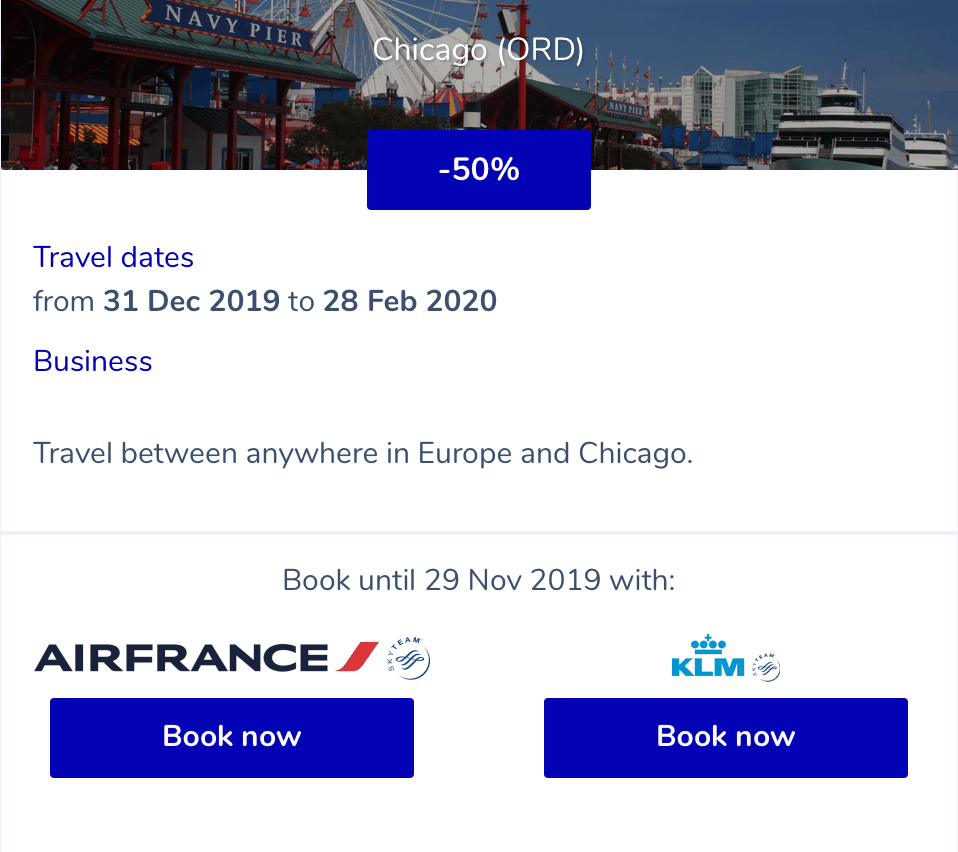The image, sourced from a website, prominently features "Chicago (ORD)" at the top. In the background, there is a scenic view of Navy Pier, showcasing a bustling attraction with a couple of large ships inviting visitors on board. Adding to the lively atmosphere is a Ferris wheel and other carnival games, giving the pier a playful vibe. A luxury apartment complex or high-end motel is visible in the distance, accentuating the skyline.

Overlaying this picturesque scene is a promotional banner. At the top of the image, set within a royal blue rectangle, is a bold "Minus 50%," capturing the viewer's attention. Below this offer, the travel dates are listed: "31 December 2019 to 28 February 2020." The term "Business" is displayed prominently in blue print.

Further details explain that the offer is available for travel between Europe and Chicago, with bookings open until 29 November 2019. Travel partnerships are highlighted, showing options to book through Air France, identified by its signature red swoosh and circle logo, or through KLM, each with a "Book Now" button in a royal blue rectangle, urging immediate action.